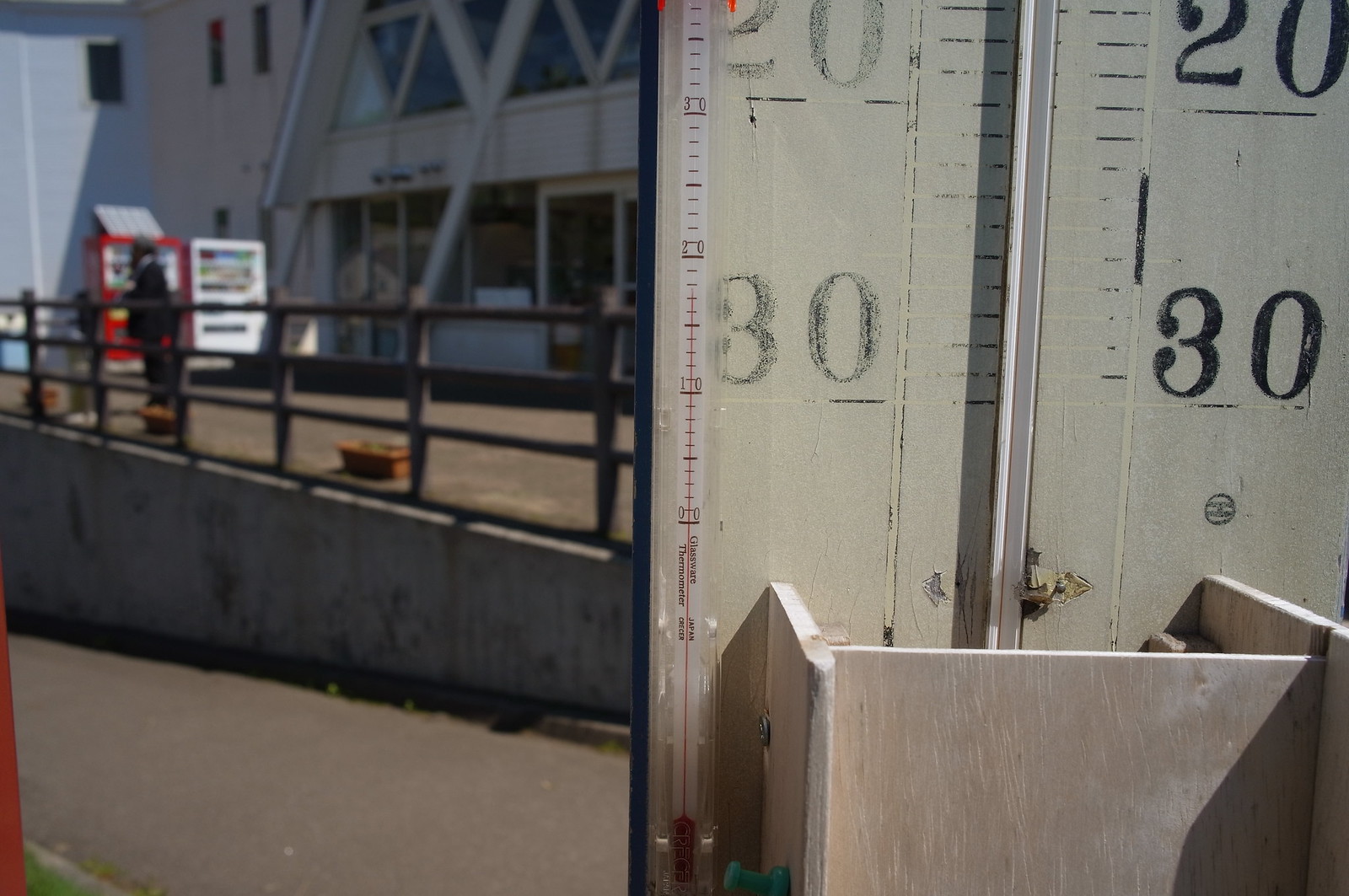A detailed outdoor photograph showcases a worn wooden temperature gauge occupying the right half of the image. The gauge, marked with black painted numbers, displays prominently: on the left side, the numbers are significantly faded, whereas on the right, they appear freshly painted and much clearer. It indicates temperatures with '30' and '20' on both sides of the gauge. Notably absent is the typical red indicator, leaving only a white bar where the indicator would normally be, suggesting that the gauge is likely non-functional.

On the left side of the image, the scene extends to include the exterior of what appears to be a commercial building, possibly a store. Nestled to the left of the store’s entrance are two vending machines—one white and one red—seemingly connected side-by-side. In front of these machines, standing along a fenced area, is a person. The fence is adorned with several terracotta pots, each containing small, barely-visible plants. The entirety of this setup—the vending machines, person, and potted plants—rests on a paved area in front of the store.